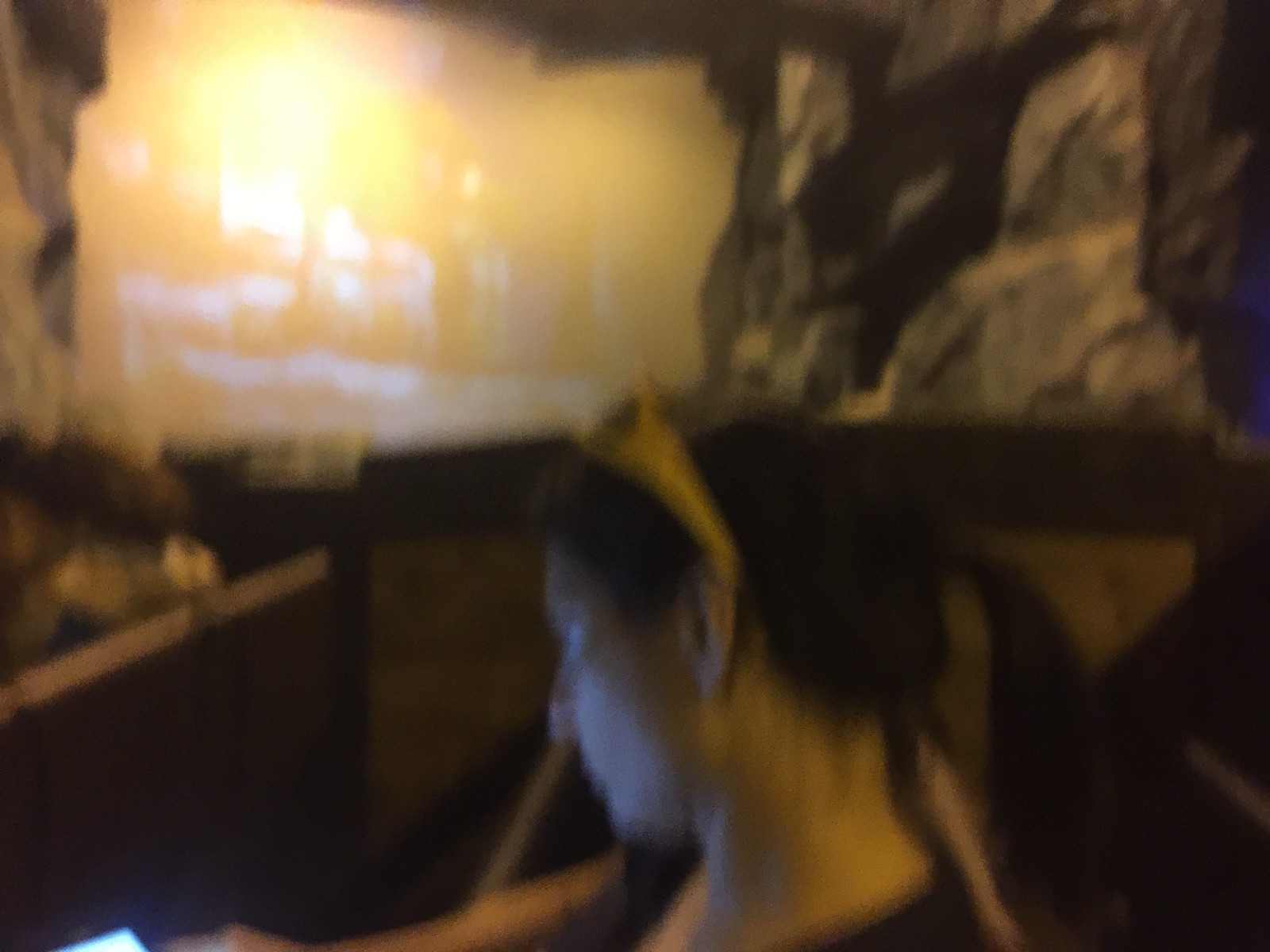In this dim and slightly blurry photograph, a woman is captured in profile while seated in what appears to be a church pew. Several rows of long benches stretch out in front of her, reinforcing the serene, contemplative setting. Her brown hair is styled in a knot atop her head, adorned with a pair of yellow plastic sunglasses resting on it. The warm glow from her cell phone illuminates her face as she looks down at the screen, suggesting she is deeply engrossed in her device. She is dressed in a simple black short-sleeve shirt. Surrounding her, a few rows ahead, are other individuals seated, visible only from the back. The background reveals a rocky wall, giving the impression that the scene might be taking place inside a natural cave. In the distance, an opening allows bright light to spill in, highlighting a building across the way and creating a striking contrast to the dim interior.